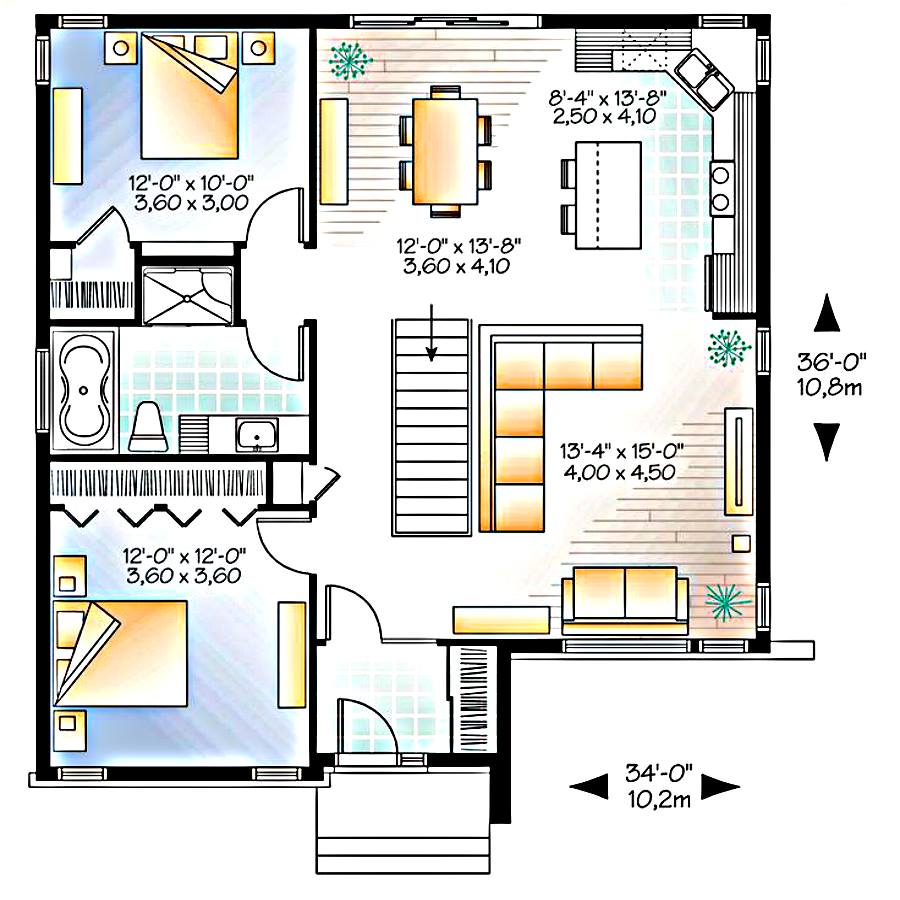This detailed floor plan is a colored sketch or CAD drawing of a two-bedroom, one-bathroom apartment viewed from a top-down perspective. The apartment layout is essentially square in shape. 

In the upper left corner, there is a master bedroom, which is illustrated in blue with a tan bed. The dimensions for the master bedroom are specified as 12 feet by 10 feet. Situated directly below this bedroom is some closet space, followed by the bathroom. The bathroom is denoted with blue tile symbols, featuring a layout where the tub is on the left, the toilet in the middle, and the sink on the right. 

Occupying the lower left corner of the apartment is another bedroom, which measures 12 feet by 12 feet, potentially making this the master bedroom instead. The bed in this room is positioned perpendicular to the left wall.

Moving to the upper right corner, we find an open-concept kitchen. The kitchen sink is set diagonally in the right corner, with the kitchen space measuring 8 feet 4 inches by 13 feet 8.5 inches. Adjacent to the kitchen, slightly to the left and near the top center of the layout, is the dining room, which measures 12 feet by 13 feet 8 inches.

Below the dining room, there is a staircase indicated on the plan. In the lower right corner, we can see the living room, furnished with an L-shaped sofa and a flat panel TV mounted on the right wall. The living room dimensions are 13 feet 4 inches by 15 feet.

Additionally, there are dimension markers along the outside edges of the square layout. On the right side, a black arrow pointing upwards and another pointing downwards indicate the wall length as 36 feet. At the lower right corner, another dimension marker shows the width of the apartment as 34 feet. All dimensions are noted in feet and inches, with their metric equivalents provided below.

This floor plan efficiently organizes the two-bedroom, one-bathroom apartment, making optimal use of the available space.